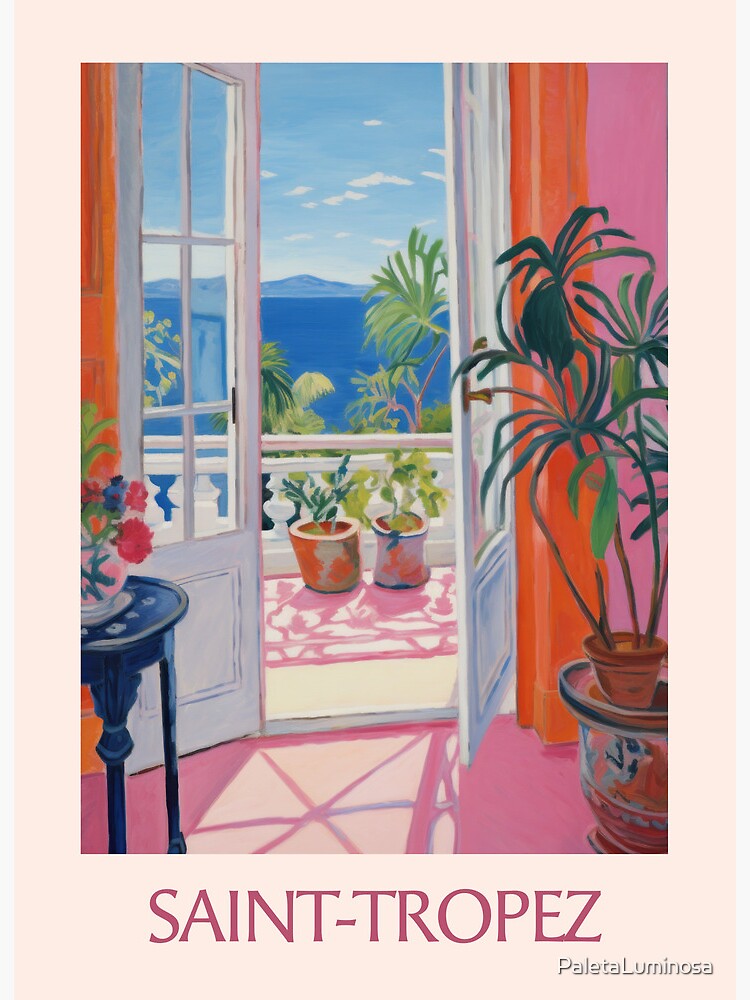The image is a vintage-style painting with pastel colors that captures the tropical charm of San Tropez. The bottom of the artwork features the inscriptions "San Tropez" in a red hue and "P-A-L-E-T-A Luminosa" in the bottom right. Dominated by pink and orange tones, the scene showcases a cozy room with double white doors opening onto a balcony. The walls and floor of the room are painted in light pink. On the left side, a table adorned with flowers complements the vibrant ambiance. Bright orange curtains frame the doors, adding a cheerful contrast. Inside the room, a small plant stands on a vase to the right. Stepping onto the balcony, the viewer is greeted by white guardrails, two potted plants, a stunning blue ocean, lush green palm trees, and a majestic mountain in the distance beneath a sky dotted with clouds. The painting's vivid colors and tropical elements evoke a serene, inviting atmosphere.